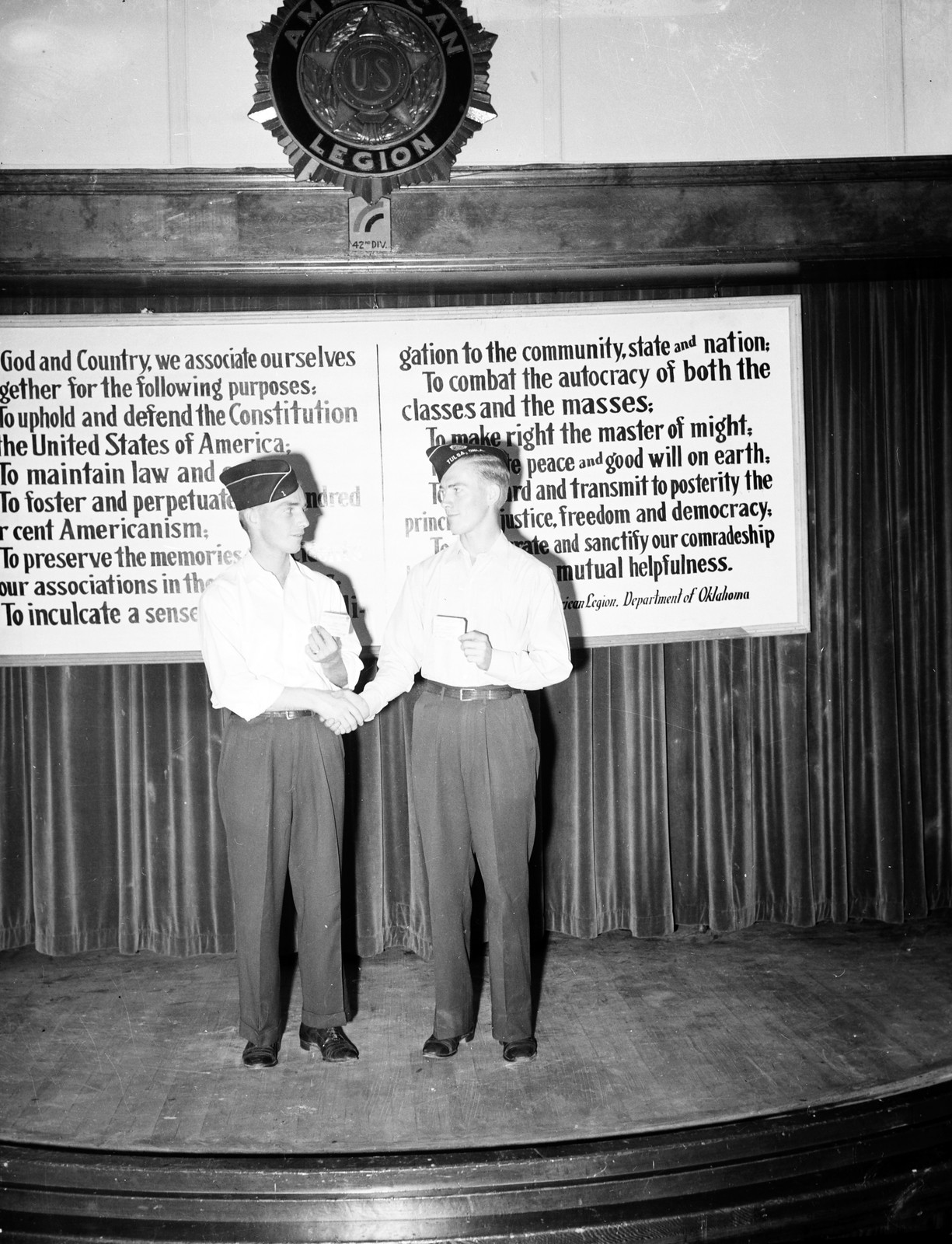This black and white, vertical rectangular photograph captures a historical moment, likely at an American Legion Hall. Two young men, dressed in identical uniforms consisting of white dress shirts, dark pants, military-style hats, and dress shoes, stand on a stage with a curtain backdrop. They are shaking hands in a formal manner, and it seems one may be presenting an award to the other. Behind them, a white plaque with black lettering is visible, just above their torsos to their heads, and a partially visible emblem reading “Legion” adorns the top of the stage. The legible text on the plaque mentions principles such as "God and country," "uphold and defend the Constitution of the United States of America," and other patriotic declarations, highlighting the American Legion's dedication to community and national service.